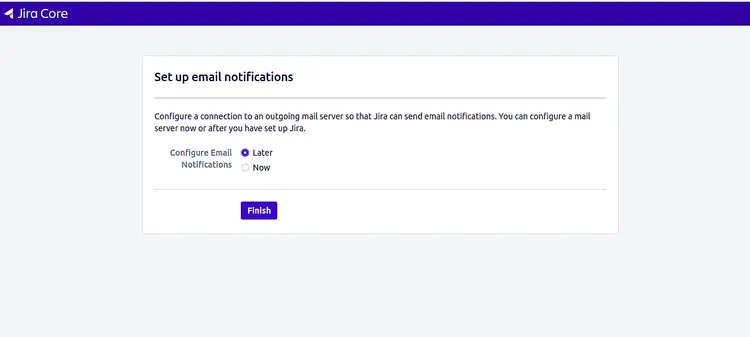The image is a detailed screenshot of the notification settings screen for a website named JiraCore, identifiable by its triangular mountain-like logo positioned at the top left corner of the screen. The logo features a peak that is slightly skewed towards the top right. The header section—which contains the logo—is shaded in purple, contrasting with the predominantly gray background of the rest of the interface.

At the top portion of the screen, large text reads "Set up email notifications," guiding users to "configure a connection to an outgoing mail server so that Jira can send email notifications." Below this, there is an instruction indicating that users can either configure the mail server immediately or defer the task until after setting up Jira.

Further down, the screen provides two options: "Configure email notifications," supported by two action buttons labeled "Later" and "Now." It appears that the "Later" option has been selected, as evidenced by its purple highlight. 

At the bottom of the screen, a prominent purple "Finish" button is present, allowing users to save their current choices and conclude the setup process.